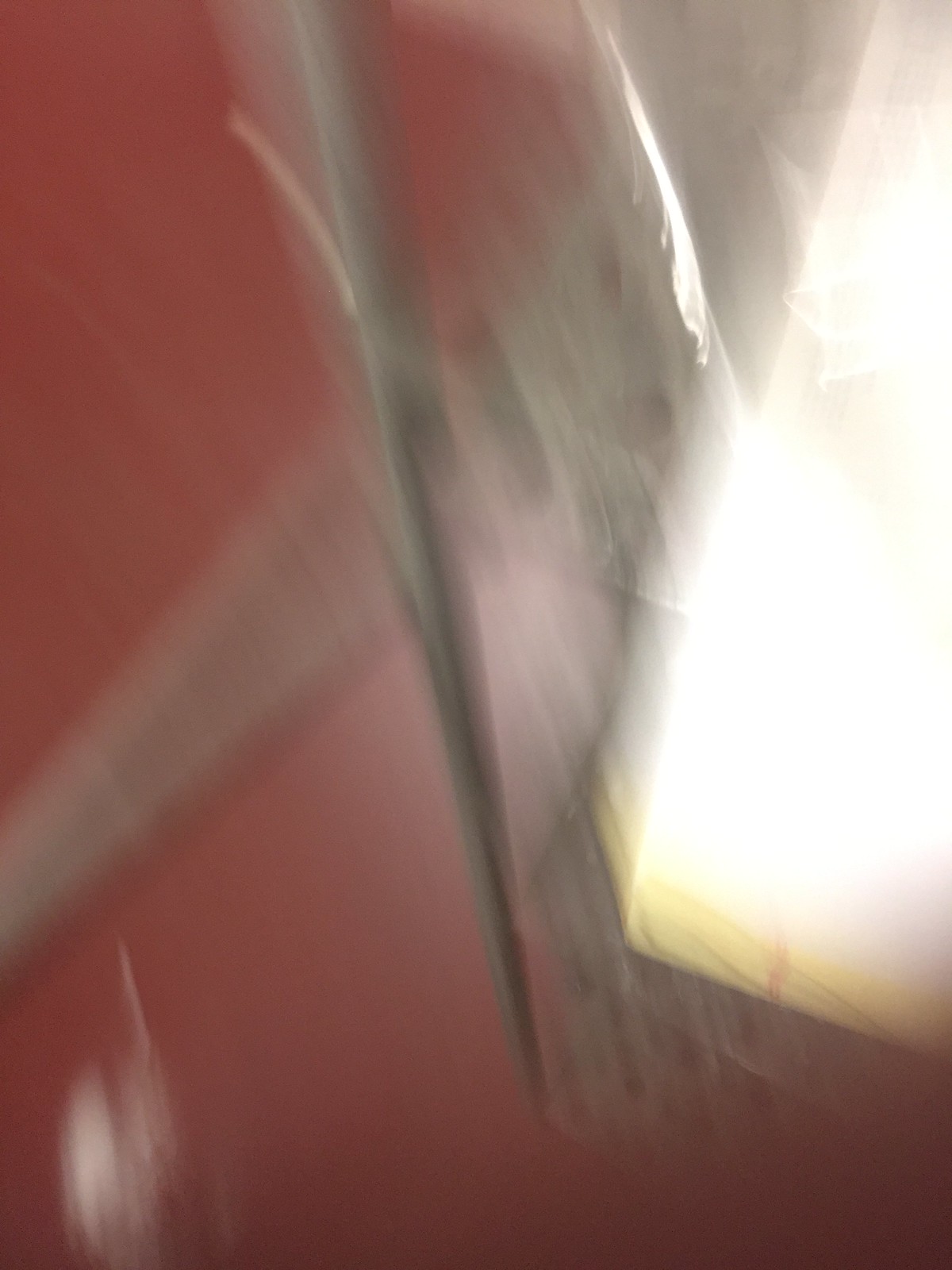This image is a very blurry photograph, likely affected by motion blur. The background is predominantly red, creating a striking contrast with a bright light or overexposed white area on the top right, which may be sunlight hitting a curtain. In the center of the image, there appears to be a clear, plastic-like object, possibly resembling a pickaxe handle protruding from the left side. Below this handle, there is a white-colored item, adding to the composition's complexity. At the bottom of the photo, lines and textures are visible, with a darker area towards the bottom right corner that hints at a black shade. Vertical, grayish striped lines are also discernible, adding to the overall visual confusion caused by the blur.